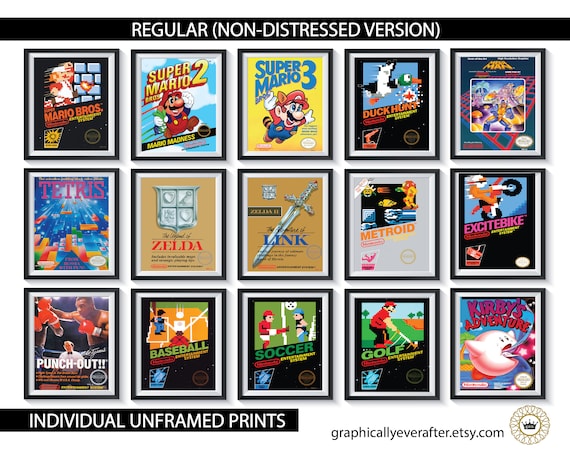This image features a collection of framed color illustrations of classic video game package covers, arranged in three rows of five. Each print is encased in a black frame with a white mat border. At the top, a black bar with white text reads "Regular Non-Distressed Version." The image includes detailed illustrations of various game covers: "Mario Brothers" with black and red lettering on a black background, "Super Mario 2" featuring a smiling Mario in his red jumpsuit, "Super Mario 3" with Mario flying against a yellow background, and "Duck Hunt." Other recognizable game covers include "Tetris," "Zelda," "Link," "Metroid," "Excitebike," "Punch-Out!!," "Baseball," "Soccer," "Golf," and "Kirby's Adventure." At the bottom left, a black bar contains white text with the phrase "Individual Unframed Prints," while on the bottom right is the text "GraphicallyEverAfter.etsy.com" beside a gold circle emblazoned with a black crown.